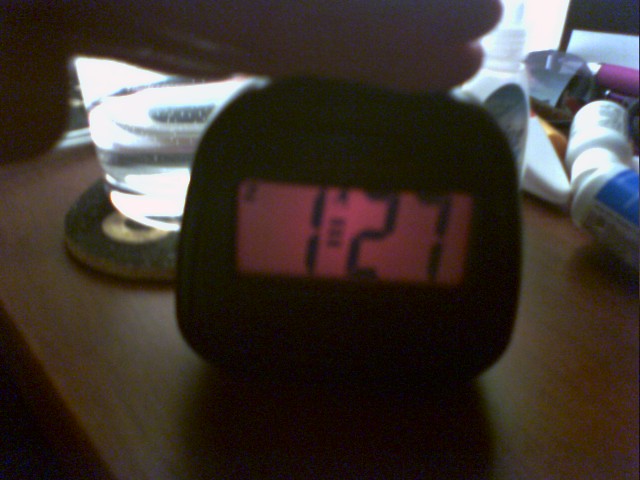The image depicts a somewhat dimly lit bedside table made of medium brown wood. In the foreground, there is a small digital clock with a dark frame and a rectangular face that has a slight pink tint, displaying the time 1:27 in black numbers. Directly behind the clock, slightly to the left, there is a glass of water placed on a thin, black and yellow coaster. Scattered around the table, particularly to the upper right corner, are several medicine or vitamin bottles, some of which are laying on their sides. One bottle with a white cap is positioned prominently, butting into another bottle with a blue label. Among the items, there's a standing bottle of either eye drops or ear drops with a white cap, and a bottle of nose spray with a dark blue label is also visible. Additionally, there are some papers with indistinct black markings and something purple positioned towards the back.